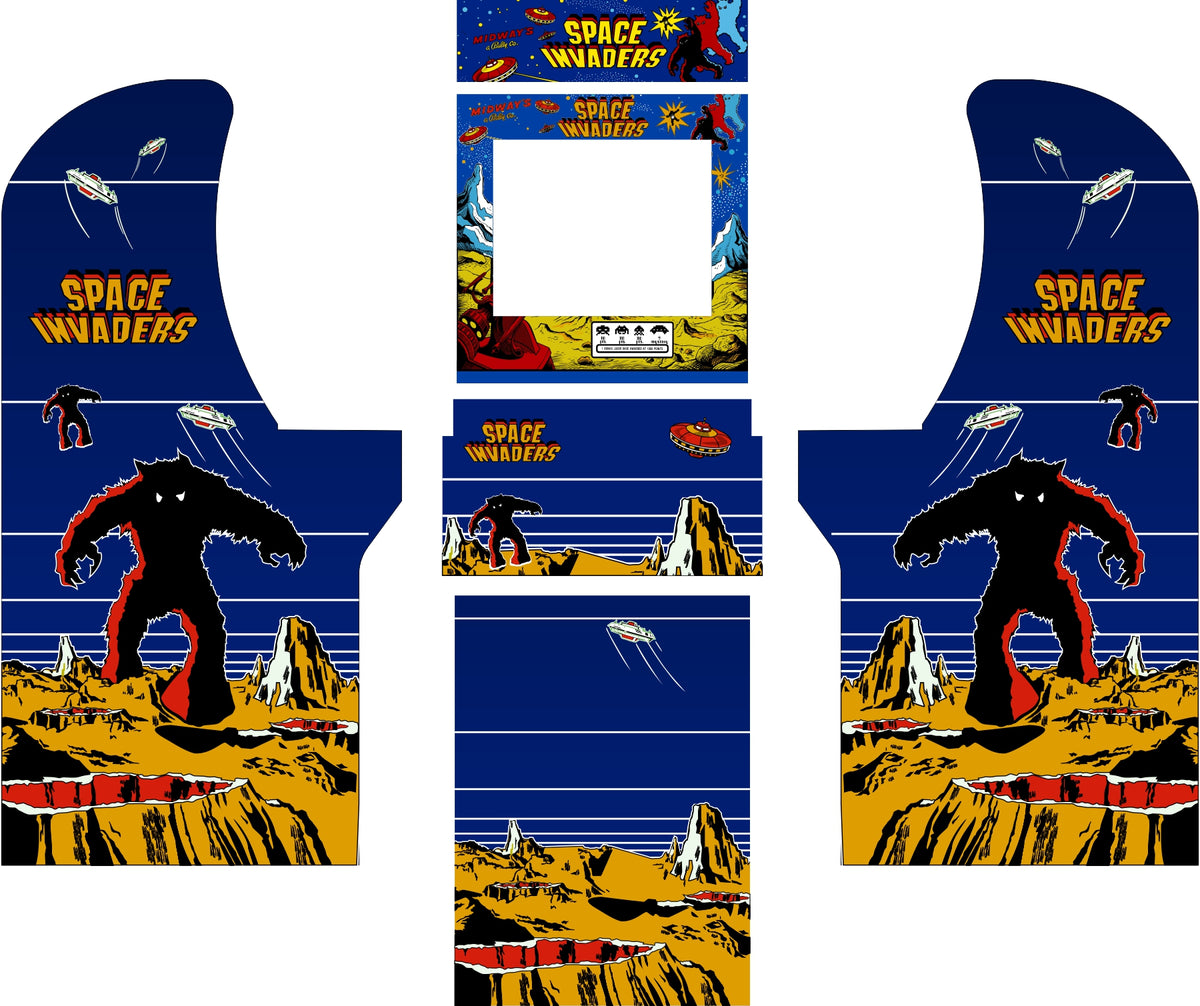The image depicts a detailed mock-up layout for the exterior graphics of a classic Space Invaders arcade game machine, displayed against a plain white background. The cut-out sections include designs for the left and right side panels, the control area, and the header and screen areas. 

Each side panel features a black humanoid-like alien creature with red outlines, white eyes, and claws, trampling across a light brown moonscape dotted with red craters. The background above the creature is blue, populated with multiple silver flying saucers. The title "Space Invaders" is prominently displayed in yellow or orange at the top of the scene.

The center section shows additional components: a square cut-out for the screen area and a rectangular section for the control panel. The imagery includes another depiction of the creature on the left, a UFO on the right, and a moonscape at the bottom. Overall, the graphics are designed to fit seamlessly on the freestanding arcade game, providing a nostalgic and vivid visual experience even in its conceptual, laid-out form.